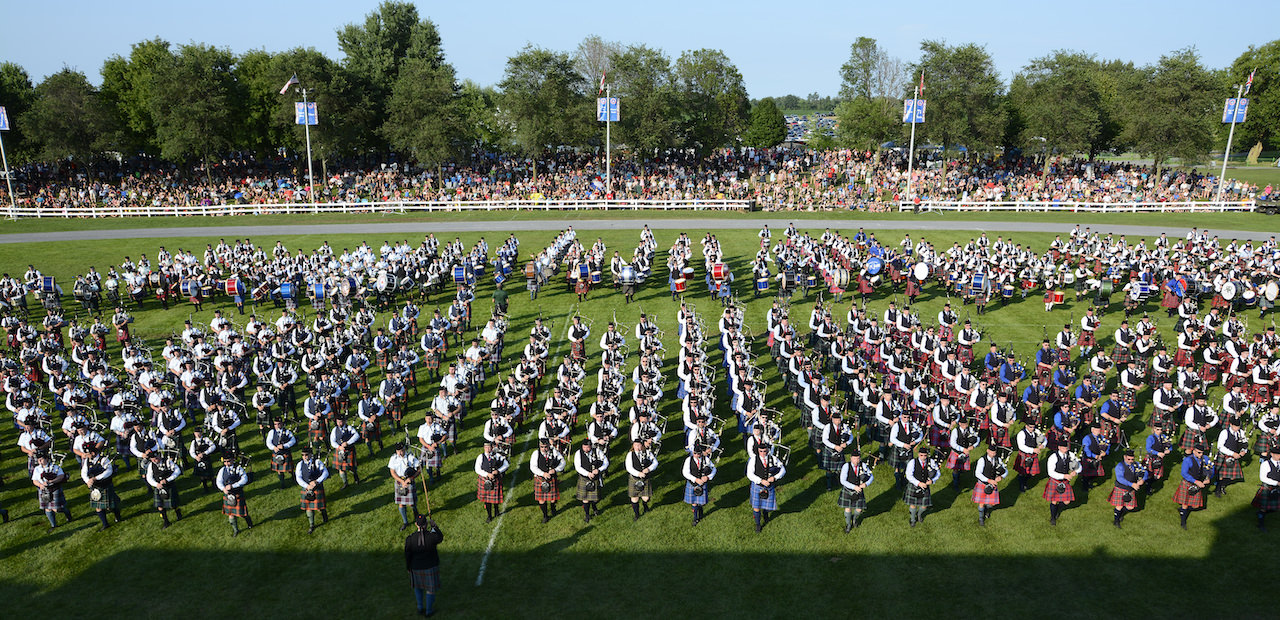This vibrant, rectangular landscape photograph taken outdoors during the daytime captures the bustling energy of the Glengarry Highland Games in Scotland. In the forefront of the image, on a lush green field, rows of predominantly men are lined up in precise formations, each group distinguished by matching kilts, white long-sleeved shirts, black vests, and black hats. All participants are playing bagpipes, holding the iconic Scottish instruments in a display of synchronized performance. The foreground's bottom left, subtly shaded, highlights the conductor orchestrating this grand spectacle.

Behind the performers, the expansive scene transitions to a running track that envelopes the field, and further back, a white fence delineates the spectator area. A dense crowd of onlookers, seated under a canopy of trees, enjoys the performance, their attention focused on the harmonious melodies of the bagpipes. Above the audience, tall banners with colorful flags stand prominently, enhancing the celebratory atmosphere. The clear blue sky overhead completes this picturesque depiction of a cultural festivity, celebrated with tradition and communal enthusiasm.